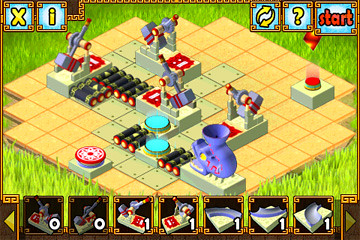This detailed caption provides a more structured and thorough description of the image mentioned:

---

A computer-generated image from a video game developer showcases a complex, tile-based game board set against a grassy background. The screen is populated with various interactive elements, including what appears to be buttons, batteries, a purple funnel, and several turquoise dots, reminiscent of components from an Erector Set. 

Prominently featured at the top of the screen are interface icons: an 'X', an 'I', a 'redo' symbol, a question mark, and the word 'Start' highlighted in red on the right-hand side. Beneath these controls are multiple tiles, each serving a unique function within the game. One tile displays "0, 0," another shows "1 left," accompanied by a hammer icon, and a third depicts a rat trap with a "1." These tiles and icons suggest a strategic puzzle element where players can place different objects to solve the maze or accomplish specific tasks.